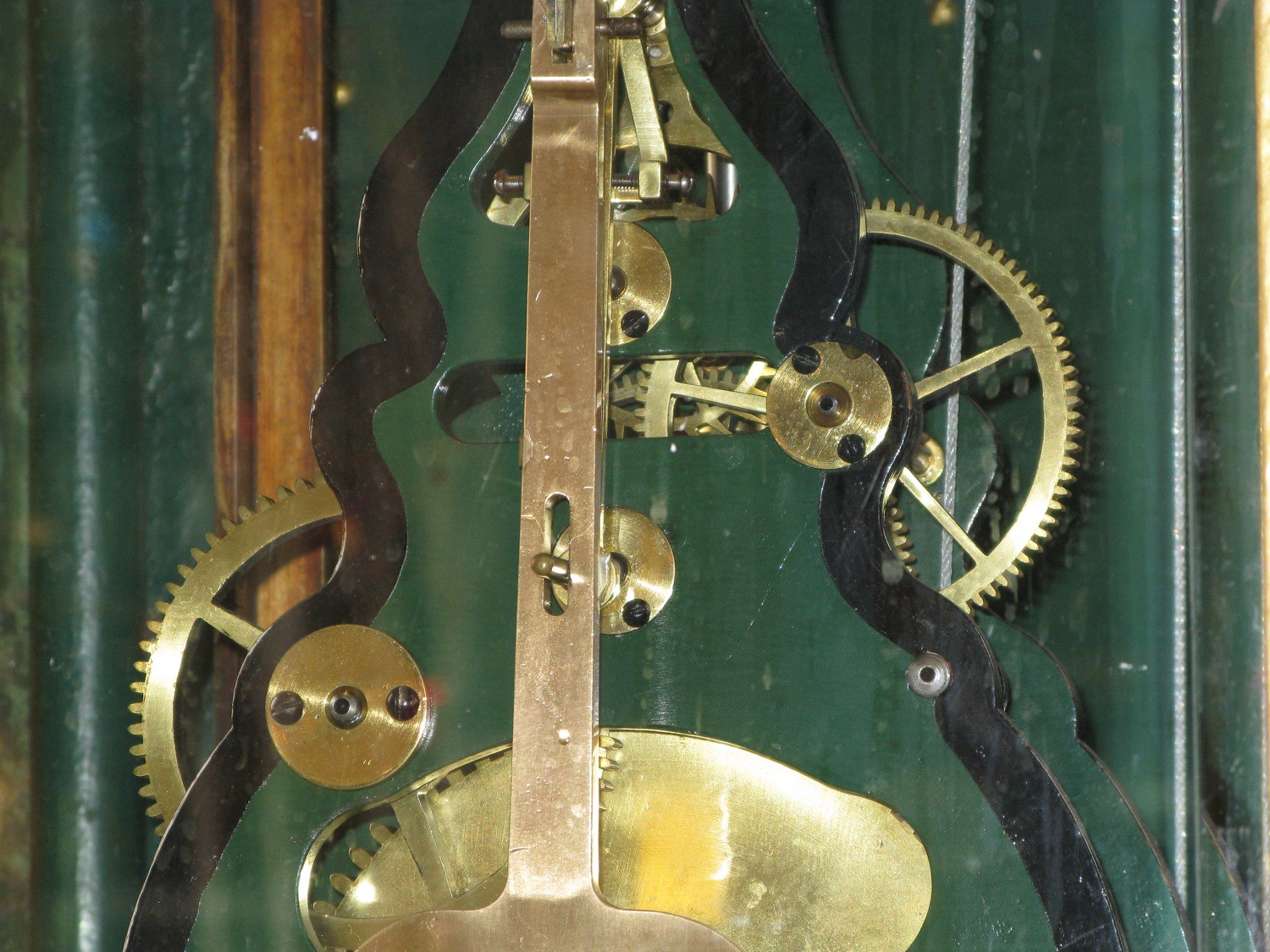The image is a detailed close-up of the inner workings of a clock, showcasing its intricate mechanical components. The background is dark green with some areas showing flaking paint and pits, which adds a textured, aged appearance. Prominently featured are various gold, brass, and silver gears—some of which are large with teeth and bracers that are rectangular in shape. Toward the top right, you can observe gold gears, while on the left, closer to the bottom, there are black, wavy metal pieces interwoven with circular gold parts. A pendulum and various brass attachments intertwine with the cogs and wheels, illustrating the complex mechanism. Additionally, you can see part of the wooden frame of the clock to the left-hand side, which is dark in color. The overall composition foregrounds the meticulous assembly of these components, presenting a captivating glimpse into the meticulous craftsmanship behind the clock's operation.